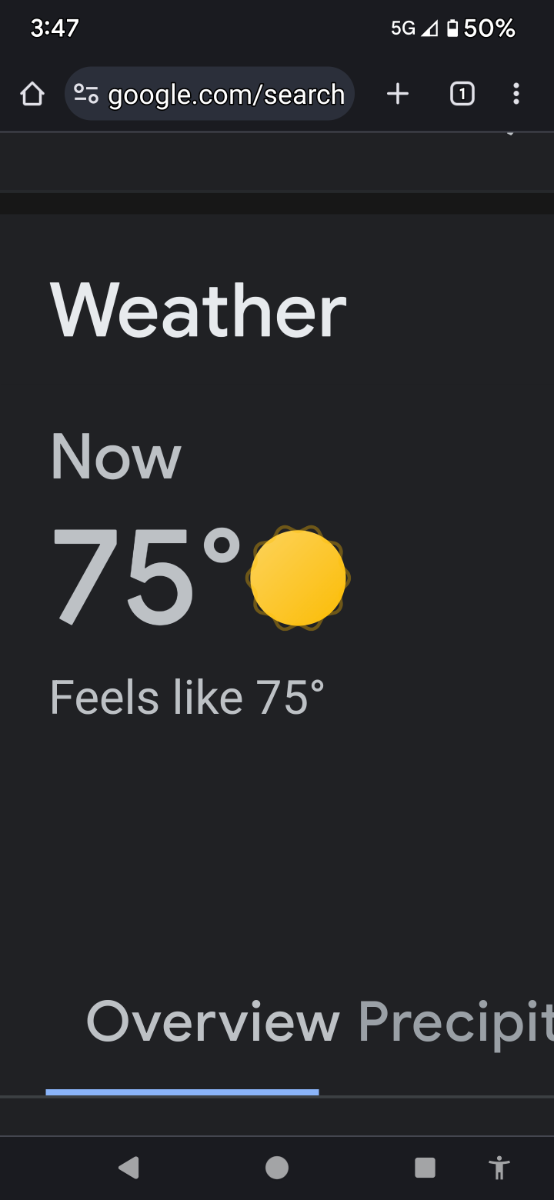A screenshot of a weather application displaying current conditions is shown. The interface has a minimalist design with a black background. At the top, the word "Weather" appears in white text. Below, "Now" is displayed in gray text followed by a larger gray text showing the temperature as "75°F." A yellow circle symbol, indicating sunny conditions with no clouds, accompanies the temperature. The phrase "Feels like 75°F" is written underneath, signifying that the perceived temperature matches the actual temperature. At the bottom, there's a section labeled "Overview" and the beginning of the word "Precipitation," which is partially truncated. The screenshot appears to be taken from a smartphone, evidenced by the on-screen navigation buttons at the bottom: the back button on the left, the home button in the center, and the recent apps button on the right. Additionally, an icon of a person with outstretched arms is visible on the far bottom right. The app does not specify the location, time, or additional weather details, providing only the essential weather information.